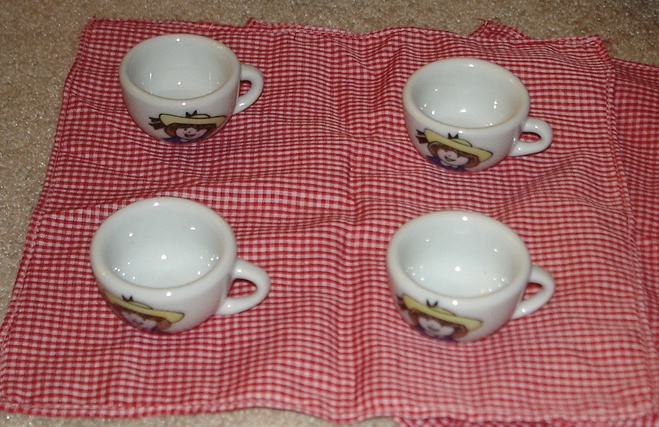This image captures a realistic, horizontally oriented photograph taken indoors. The scene is set on a light tan carpet that forms the background. In the center of this background, there's a red and white checkered cloth, possibly a tablecloth or placemat. Arranged on this cloth are four shiny, child-sized ceramic teacups, each turned so that their handles point to the right. The teacups feature a hand-drawn, cartoon character—Madeline, known from books, movies, and cartoons—on their fronts. Madeline is depicted with red hair, wearing a yellow sun hat adorned with a black bow, and dressed in a blue, white-collared dress. The overhead lights reflect off the glossy surfaces of the cups, adding a touch of brightness and emphasizing their ceramic finish.